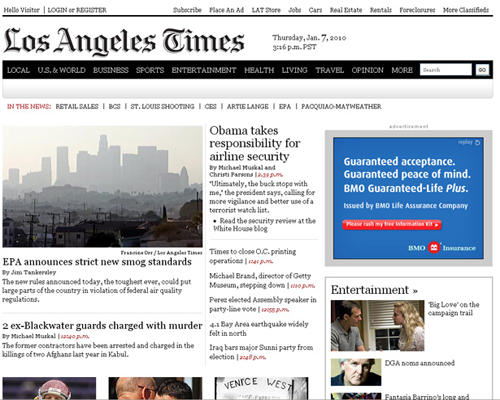This screen capture appears to be from the Los Angeles Times Archive on a white background with predominantly black text, interspersed with some red text. At the top, there is a thin black line above a navigation bar that reads, "Hello visitor, log in and register, subscribe, place an ad, LAT share, jobs, cars, real estate, rentals, foreclosures, more classifieds." 

The page is identified as belonging to the Los Angeles Times, dated Thursday, January 7, 2010, at 3:16 p.m. PST. Below another thin black line, white text on a black background categorizes content into sections: "local, US and world, business, sports, entertainment, health, living, travel, opinion, and more." A white search box accompanied by a "go" button is visible.

The main body of the page showcases a series of articles under the section "In the News," listing topics such as "retail sales, St. Louis shooting, CBS, Artie Lang, EPA, Paquiao Mayweather." An image of a foggy downtown cityscape accompanies an article titled "EPA announces strict new smog standards," followed by another headline stating, "2x Blackwater guards charged with murder."

Multiple other headlines are partially visible, including "Obama takes responsibility for airline security," "Time to close OC printing operations," references to museums, a speaker, a Bay Area earthquake, and Iraqi elections. 

There is a blue advertisement with white and red text stating, "Guaranteed acceptance, guaranteed peace of mind, BMO guaranteed life plus," and an entertainment section with partially discernible titles such as, "Big Love on the campaign trail," "DGA NOMS announced," and "Fantasia Burrino’s long," before cutting off.